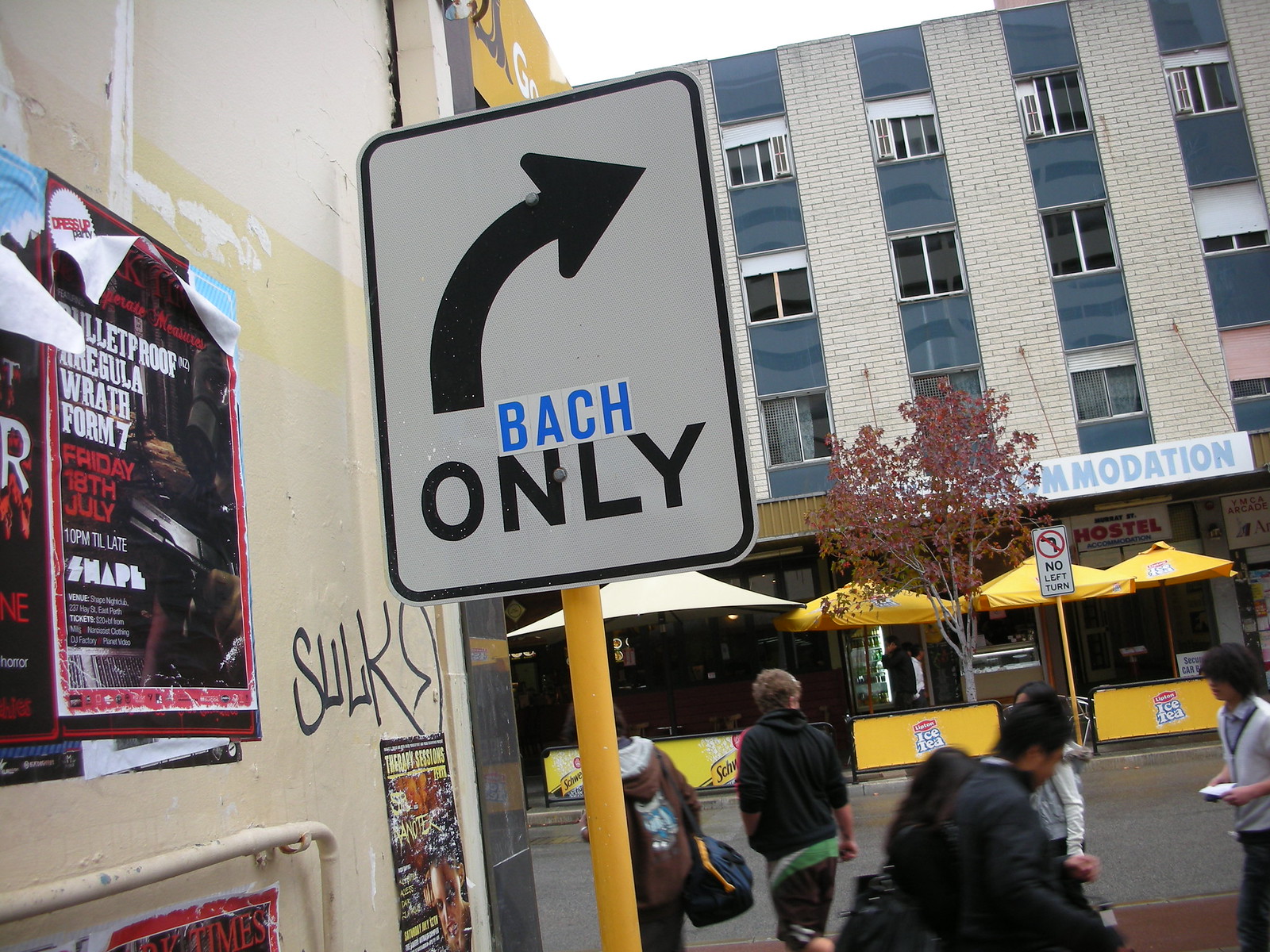The image captures a bustling city street scene with the focal point being a prominent street sign in the center. The street sign, mounted on a slightly tilted yellow pole, has a tall rectangular shape with rounded corners, featuring a white background, a curved arrow pointing towards the upper right, and the word "only" below the arrow. Superimposed on the sign is a blue-lettered sticker spelling "BACH," which contrasts with the black text of the original sign. The background reveals a mix of urban elements: on the left, the wall of a building adorned with various posters and graffiti; and directly behind the sign, a multi-story building with distinct blue windows and a ground-floor restaurant marked by yellow umbrellas and tables. The scene is further animated by people walking in various directions, adding to the dynamic city atmosphere.